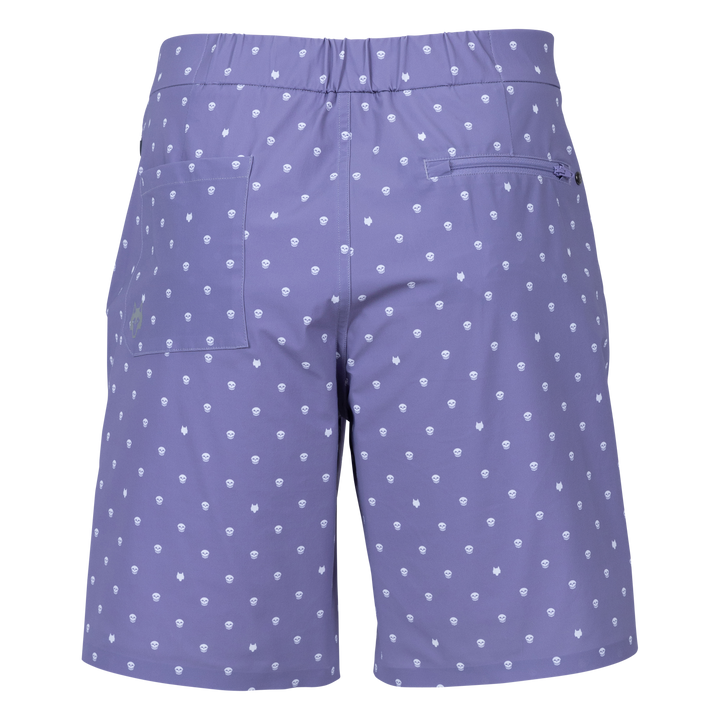Set against a completely white background is a pair of long shorts that are a purplish-blue color, potentially verging more on a purple hue. The shorts extend down to about knee level and are viewed from the back, revealing two distinctive back pockets. On the left side, there is a regular, deep pocket, while the right side features a pocket with a matching colored zipper and zipper teeth. An elastic waistband at the top enhances comfort. Intricately decorating the entire fabric are small, evenly spaced white skeleton heads and white fox head patterns, scattered thoughtfully across the shorts. Additionally, a noticeable seam is present at the waist, and a small black button is situated on the right side, adding a subtle yet functional detail to the overall design.